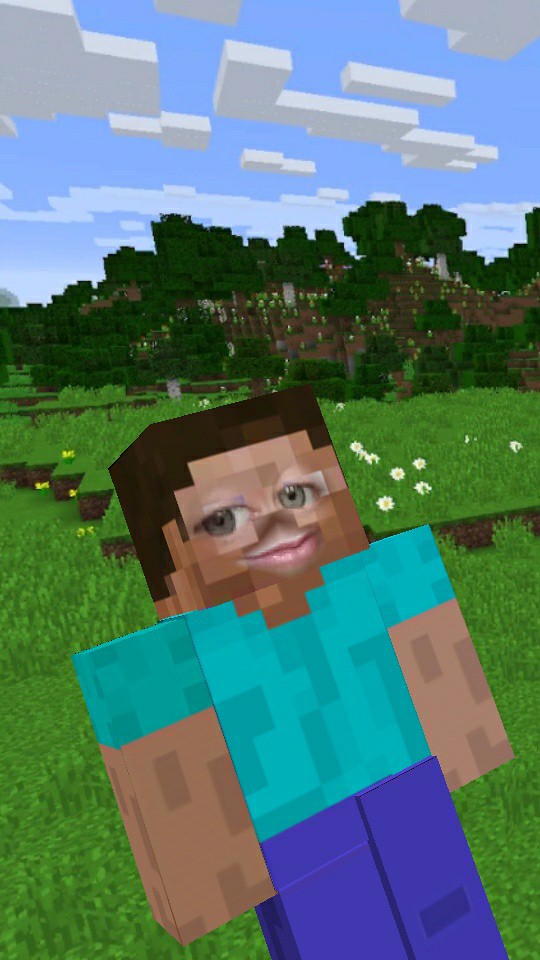This is a detailed illustration of a seemingly animated character, crafted in a distinct cube-like design. The character, which appears to be either a man or a boy, is composed entirely of squares and rectangular shapes. His head is perfectly square, and he is adorned in a light blue short-sleeved t-shirt. The continuation of the geometric theme is evident in his rectangular arms and the long, rectangular blue pants he wears. The backdrop of the image features a lush landscape with abundant green grass, studded with small, white flowers. In the distance, there is a gentle hill dotted with trees, further emphasizing the scenic, natural setting. The entire scene presents a unique blend of geometric character design set against a richly textured, natural environment.